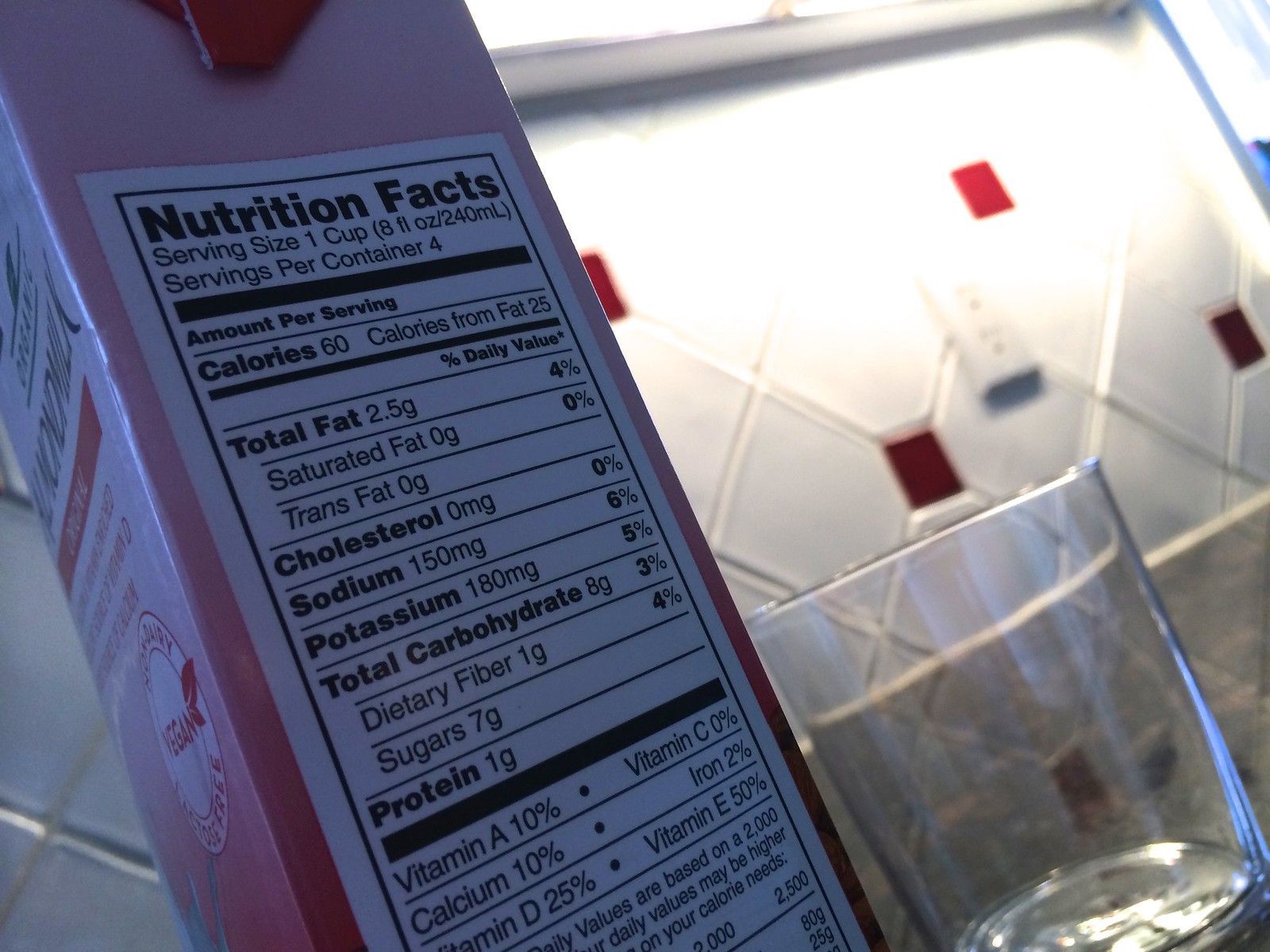The image portrays a light pink and whitish cardboard wax container of almond milk positioned on a counter in front of a tile wall adorned with brown and red dots, alongside an electrical outlet. The carton features a detailed Nutrition Facts panel indicating a serving size of 1 cup (8 fluid ounces) with 4 servings per container. Each serving contains 60 calories, 2.5 grams of fat, no cholesterol, 150 milligrams of sodium, 8 grams of carbohydrates (comprising 1 gram of fiber and 7 grams of sugar), and 1 gram of protein. The vitamin content includes 10% Vitamin A, 10% calcium, 25% Vitamin D, 2% iron, and 50% Vitamin E. The panel is presented in black print on a white background. Also, 180 milligrams of potassium are noted. Next to the carton is an empty, clear, short round glass. The front of the container displays a partially visible design, including a round circle icon which resembles an insect and is brownish-red in color.